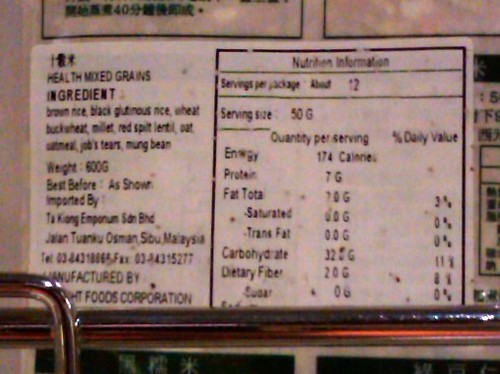This detailed close-up image shows the ingredients list label of a product named "Health Mixed Grains." The label, presented predominantly in black text on a white background, specifies the ingredients as brown rice, black glutinous rice, wheat, buckwheat, millet, red split lentil, oat, oatmeal, Job's Tears, and mung bean. The product weight is clearly listed as 600 grams, and the best before date is mentioned but not specified in the image. 

The label indicates that the product is imported by an entity located at Tay Keong Emporium, Jalan Tuanku Osman, Cebu, Malaysia. However, parts of the manufacturer's details are obscured, only revealing "Foods Corporation."

To the right of the ingredients list, there is a section dedicated to nutrition information. This section notes that there are approximately 12 servings per package, with each serving size being 50 grams. The nutritional breakdown per serving includes 174 calories, 7 grams of protein, and a total fat amount that includes subcategories of saturated and trans fats—though the exact figures for these, as well as for carbohydrates, dietary fiber, and sugar, are not legible due to print quality issues. The corresponding daily value percentages are also listed but are difficult to read.

The bottom of the image features a metal railing beneath the label.